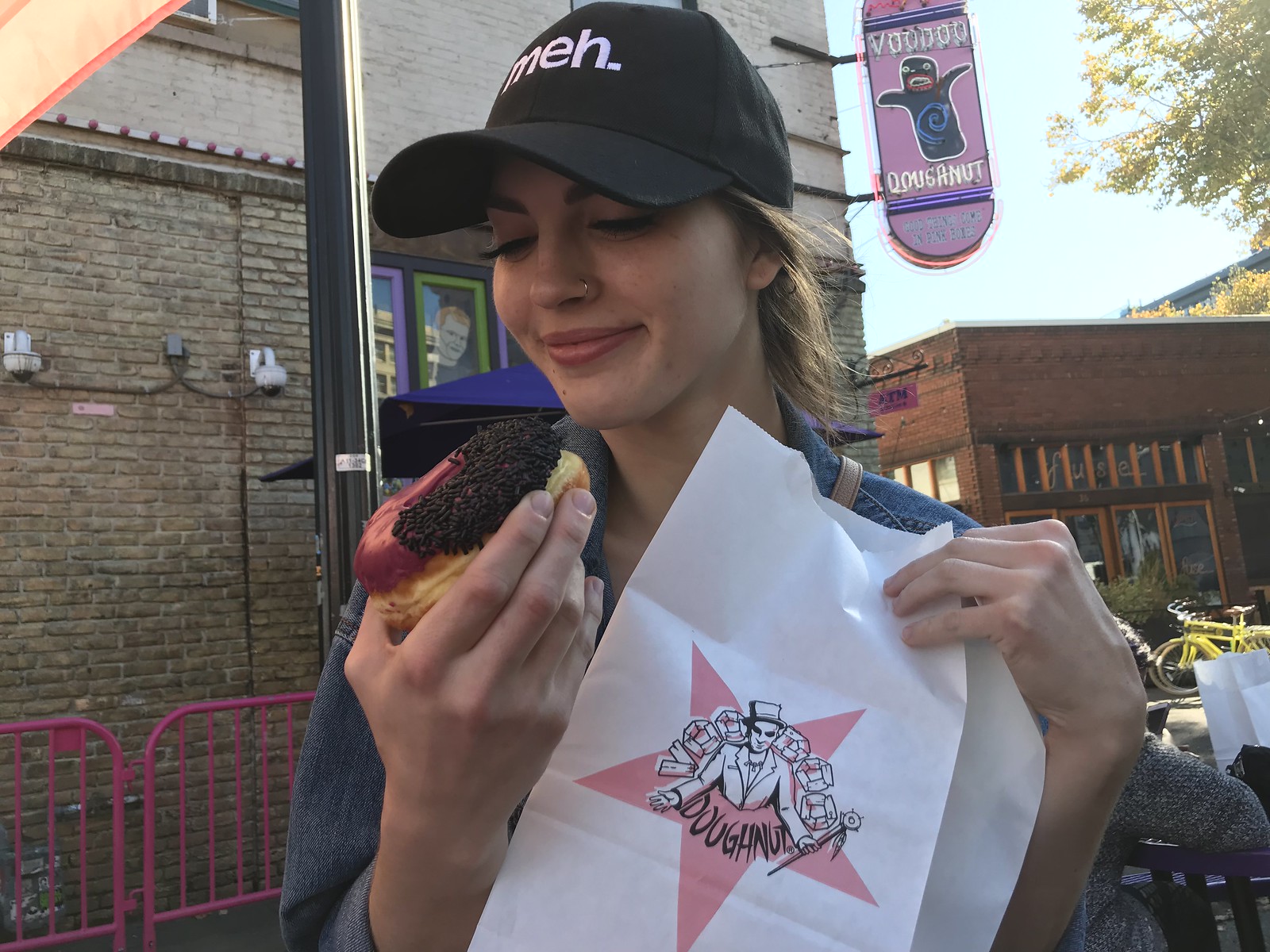In this vibrant outdoor color photograph taken during the daytime, a young girl, approximately 16 or 17 years old, is captured in profile. She has ash blonde hair peeking out from under a large black baseball cap that features the white lettering "M-E-H." A delicate smile graces her face, marked by a nose ring on her left nostril. Her head is tilted towards her right hand, where she holds a donut adorned with red strawberry frosting and chocolate sprinkles on one half. Her body is oriented towards the camera, indicating a candid moment likely shared with a friend.

In her left hand, she holds up a white paper bag, angled such that it partially covers her torso. The bag displays an emblem featuring a pink star, a black and white line drawing of a man wearing a top hat and suit, and text that likely says "donut," although the lettering is somewhat unclear. This bag appears to have been purchased from the store behind her.

The background reveals a multi-story, brick building with a neon sign reading "Voodoo Donut" to the right, hinting at the whimsical and popular establishment she just visited. A tree and a portion of the sky occupy the upper right corner, adding to the natural setting of this delightful and detailed moment.